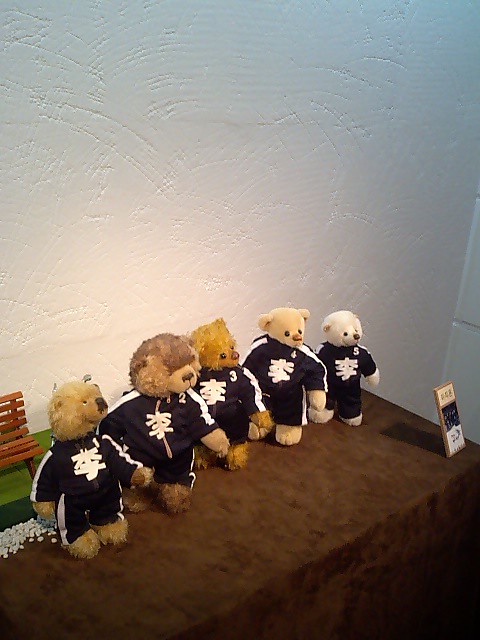This indoor photograph captures a whimsical display of five teddy bears neatly arranged on a table draped in a chocolate brown fabric tablecloth. The setting is against a white, imperfectly painted wall showing scratch lines and engravings. Each teddy bear is dressed in an identical black tracksuit with white stripes down the arms and legs, marked with a large white Asian character at the center of their chests. The bears are sequentially numbered from 1 to 5. 

Starting from the left, the first bear is beige with a black nose. The second bear is a chocolate brown with lighter fur around its snout and cheeks. The third bear, marked with the number 3, features a golden, curly fur. The fourth bear, bearing the number 4, is an off-white or tan color with a dark nose. The fifth, smallest bear, numbered 5, has a smooth, white fur accented with pink in its ears and a dark nose.

On the right side of the table, there is a small, angular sign or picture frame casting a shadow. Behind the bears to the left, there is a small, partially visible red wooden park bench, seemingly designed for dolls or stuffed animals, accompanied by white pebbles and a green felt surface.

The dimly lit photo emphasizes the details and uniforms of the bears, evoking a sense of organized playfulness, possibly suggesting a themed collectible display.